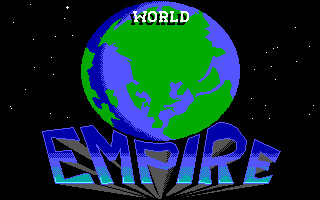This is a detailed poster portraying a stylized illustration of Earth set against a backdrop of a starry sky. The artwork is a drawing, with the Earth depicted as a perfect circle rather than the usual oval shape. The landmasses on the globe are shaded in a deep green, while the oceans are rendered in a rich purple hue.

Prominently overlaying the globe is the word "WORLD" written in bold white letters. Below the globe, the word "EMPIRE" is artistically arranged, with the characters "M-P-I" appearing to sag under the weight of the Earth, creating a sense of heaviness. The word "EMPIRE" is designed in a 3D effect, making it seem as though it is extending from the background towards the viewer. The overall effect is a visually striking and imaginative representation of a world globe, evoking a sense of grandeur and weight.